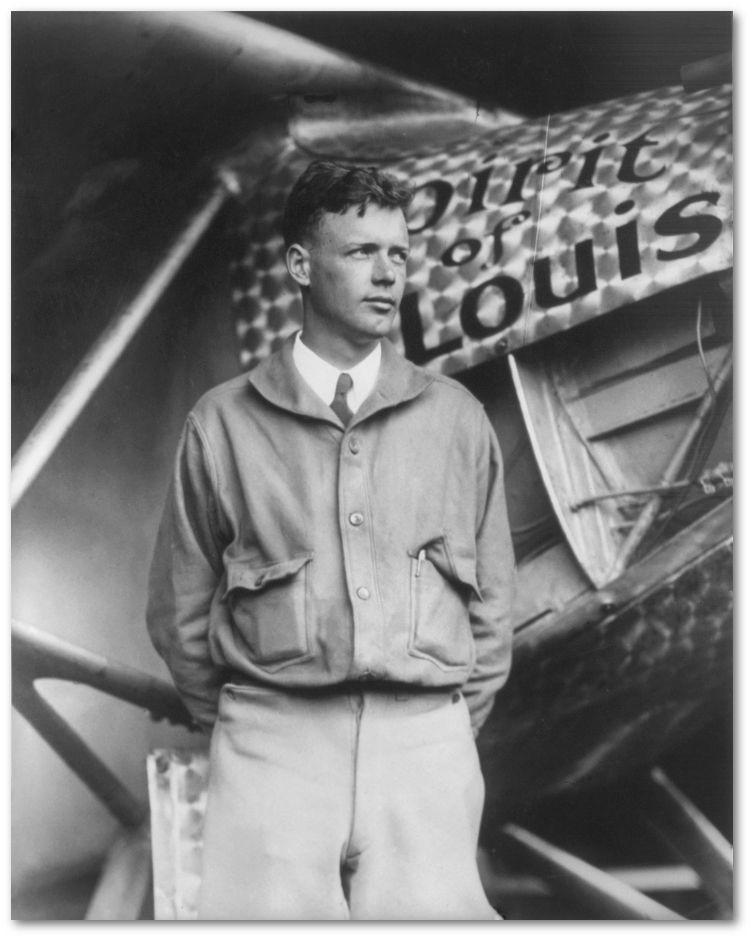In this black and white photograph, a young Charles Lindbergh stands pensively in front of his historic airplane, the Spirit of St. Louis. Lindbergh, with a slight smirk, gazes off to his left. He is dressed in an aviator jacket over a button-down shirt and a black tie, paired with light-colored pants. His hands are folded behind his back, adding to his contemplative pose. The plane, prominently featuring a smudged metallic design, occupies the background with its nose and stabilizing rods in clear view. The distinct label on the plane, partially obscured by Lindbergh’s head, reads “Spirit of St. Louis.” The background contrasts with darker shading on the upper right and bottom right corners, adding depth to the photograph where the left side remains more clear and gray. This atmospheric image captures a significant moment, highlighting both the aviator and his legendary aircraft.